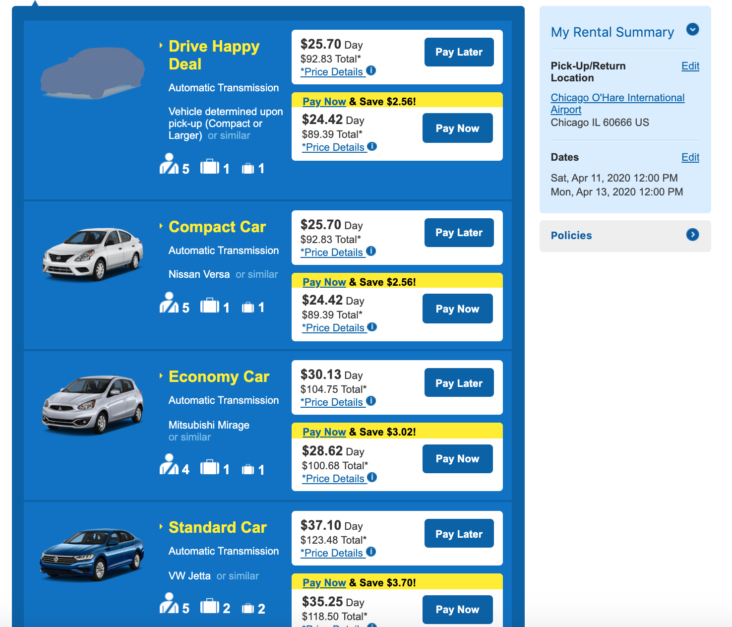**Detailed Caption:**

The image features a detailed advertisement for car rental deals. On the left-hand side, there is a dark blue rectangle with a lighter blue rectangle inside it, showcasing the outline of a car. Adjacent to the car outline, gray and white, and yellow text reads, "Drive Happy Deal." Below this, white text states, "Automatic transmission vehicle determined upon pickup. Compact or larger."

On the right-hand side, there is a vertical arrangement of pricing options within several sections. At the top, there are two white squares outlined in yellow. One square has the text "Pay Later" and the price "$25.70 a day," while the other square reads "Pay Now" with a price of "$24.42 a day."

Below these options, the next section features a white car labeled "Compact Car," with the pricing options "$25.70 a day" for pay later, or "$24.24 a day" for pay now. Beneath this, another option displays a gray car labeled "Economy Car," with pricing of "$30.13 a day" for pay later and "$28.26 a day" for pay now.

Further down, a blue car resembling a Volkswagen is labeled "Standard Car." Its rental options are priced at "$37.10 a day" for pay later and "$35.25 a day" for pay now.

On the far right side of the image, inside a bluish box with blue text, there's a section titled "My Rental Summary." The black font states the "Pickup/Return Location: Chicago O'Hare International." The blue text below specifies the rental dates as Saturday, April 11, 2020, through Monday, August 13, 2020. However, it's noted that the dates seem unlikely due to the COVID-19 pandemic occurring at that time.